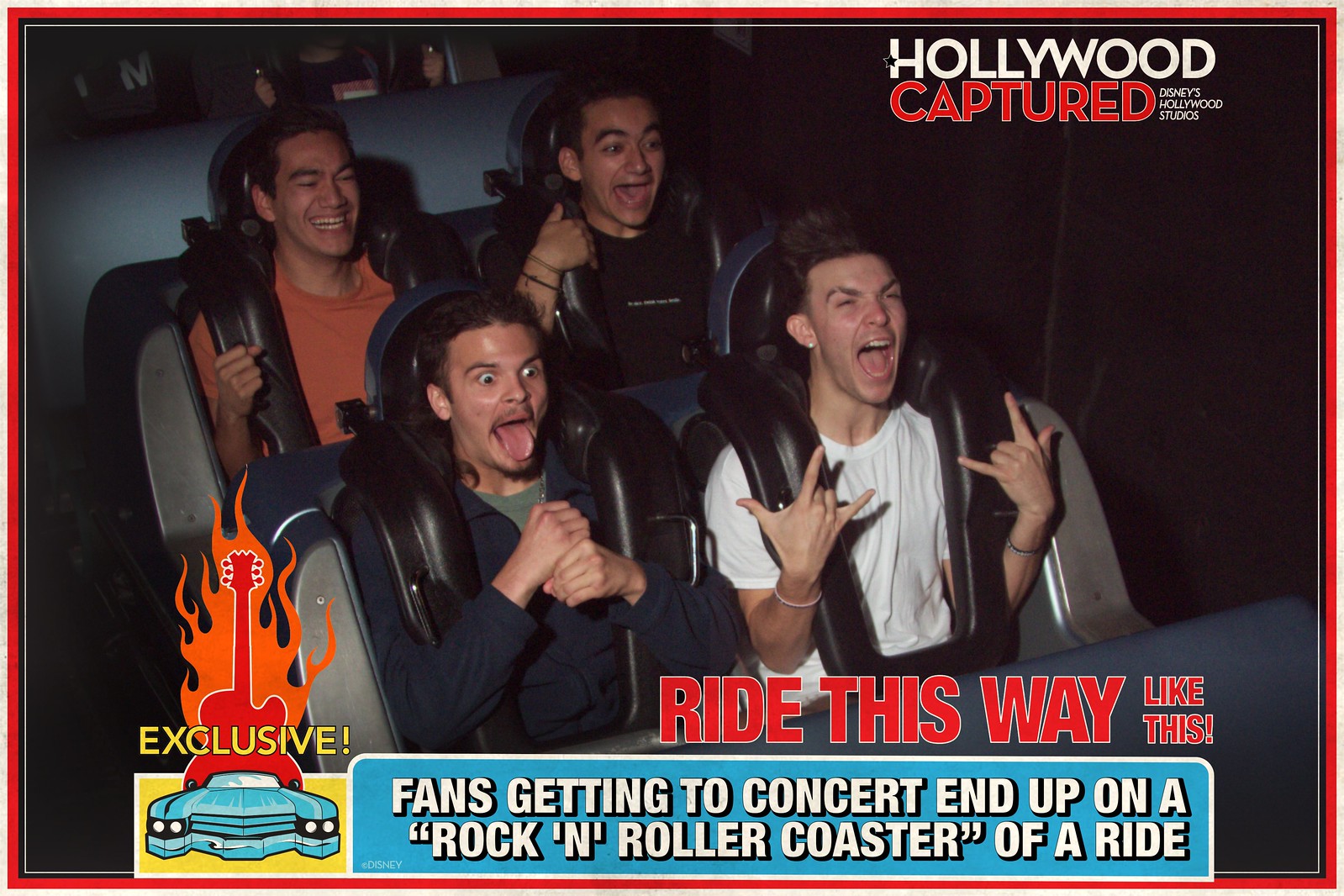The image depicts a thrilling moment captured on a roller coaster ride. Four male passengers are visibly excited as they experience the rush: one in the front right seat flashes a rock hand gesture with his mouth wide open in a scream, while the passenger next to him shows clenched fists with his tongue out. The two men behind them display expressions of pure exhilaration, one holding onto his harness with a smile, and the other with his mouth agape. 

This photo, framed with a red border, features notable text elements: at the top right, "HOLLYWOOD" appears in white all-caps, followed by "CAPTURED" in red all-caps. Directly below this, in smaller white text, the phrase "Disney's Hollywood Studios" is included. At the bottom right, a bold red banner reads, "RIDE THIS WAY LIKE THIS!" and beneath it, a blue rectangle pops with the message, "FANS GETTING TO CONCERT END UP ON A ‘ROCKIN' ROLLER COASTER’ OF A RIDE." To the left of this message, an image of a blue Cadillac and a flaming red guitar, labeled "EXCLUSIVE" in yellow all-caps, adds to the electrifying atmosphere.